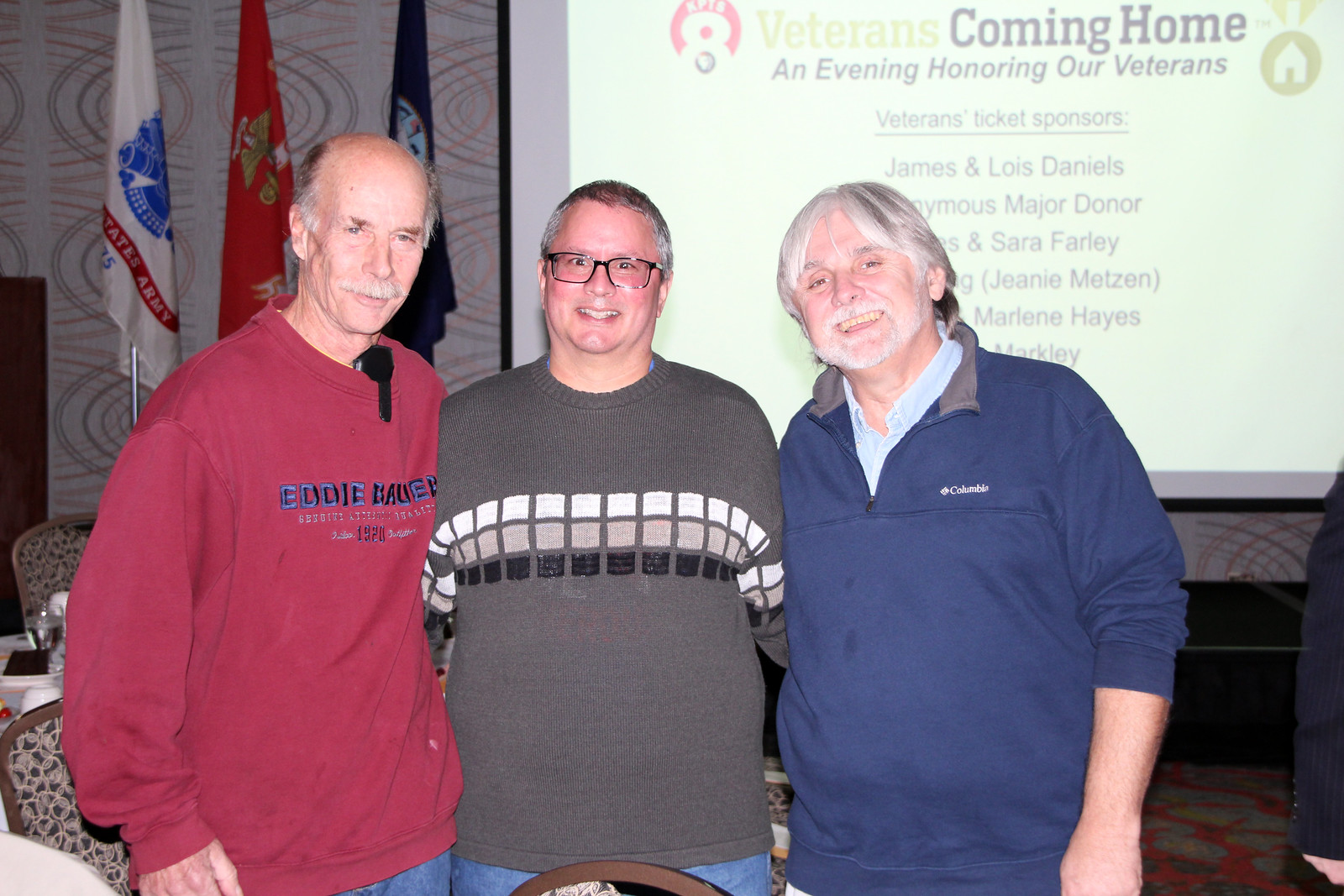Three men stand shoulder-to-shoulder, with their arms around each other's backs, smiling at the camera in front of a patterned wall adorned with three flags. The man on the left, an older individual with a gray mustache and balding head, is dressed in a large red sweatshirt that reads "Eddie Bauer" in blue lettering. The middle man, younger and bearded, wears glasses and a long-sleeve brown sweater featuring a pattern of white, tan, and black squares. The man on the right sports long white hair and dons a blue fleece pullover with a Columbia logo over a blue collared shirt. Behind them, on the right side of the frame, a projected PowerPoint slide with the text "Veterans Coming Home: An Event Honoring Our Veterans" is visible, along with a list titled "Veterans Ticket Sponsors," which includes names such as James and Lois Daniels, Major Donner, Sarah Farley, Jenny Metzen, Marlene Hayes, and Mark Lee.